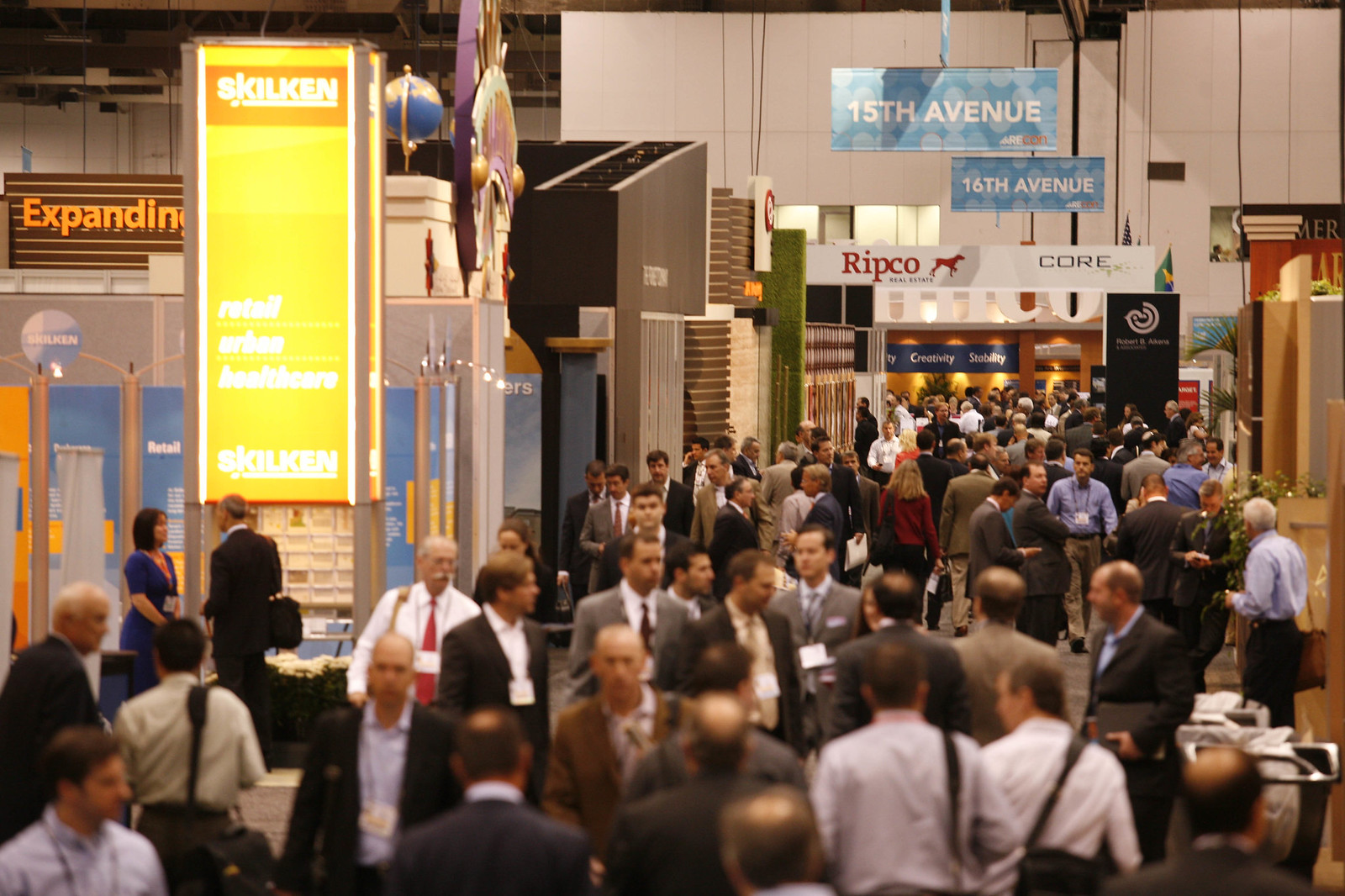The image depicts a bustling indoor professional event or conference, with a large crowd of approximately 100 people, predominantly men in business professional attire such as suits, tuxedos, and dress shirts. The scene is anchored by blue signs hanging from the ceiling that read "15th Avenue" and "16th Avenue" in white text, accompanied by a logo in the corner. In addition to these signs, various advertisements and booths can be seen throughout the venue. On the left side, an orange sign reads "Expanding," while the middle background features blue signs with the words "Creativity" and "Stability" in white text, and red text spelling out "Ripco" alongside "Core" in black. To the right, a black sign prominently displays the name "Robert B. Atkins." A notable element is a single woman in a blue dress, standing out amidst the sea of well-dressed men. The crowd converges towards the center-right of the image, suggesting a point of interest or a focal area in the conference filled with anticipation.